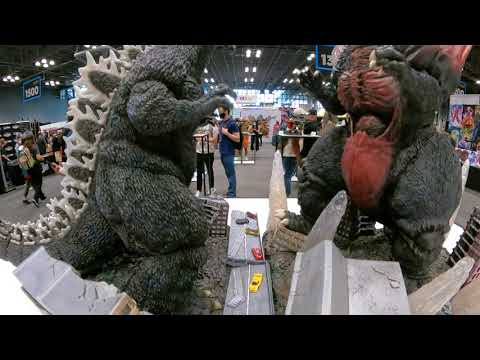The image captures the bustling atmosphere of a large convention center filled with numerous booths, exhibitors, and crowds of people. Dominating the center of the photograph is a detailed diorama depicting two colossal Godzilla-like creatures locked in combat. Both sculptures are positioned on their hind legs, with one creature facing sideways to the right and the other front-facing, showcasing its red body with white claws and distinctively chunky thighs. The scene at the base of this display is a meticulously crafted miniature urban disaster, featuring cracked roads, scattered toy cars in various colors (red, yellow, blue, black), half-destroyed buildings, and crystal spikes emerging from the ground. The ceiling of the convention hall is lined with lights, and suspended signs displaying numbers like 1500 and 1300 can be seen in the background. Beyond the central display, the image reveals a vast open space with numerous booths and tables where attendees are gathered, creating a lively, vibrant environment indicative of a large-scale convention.